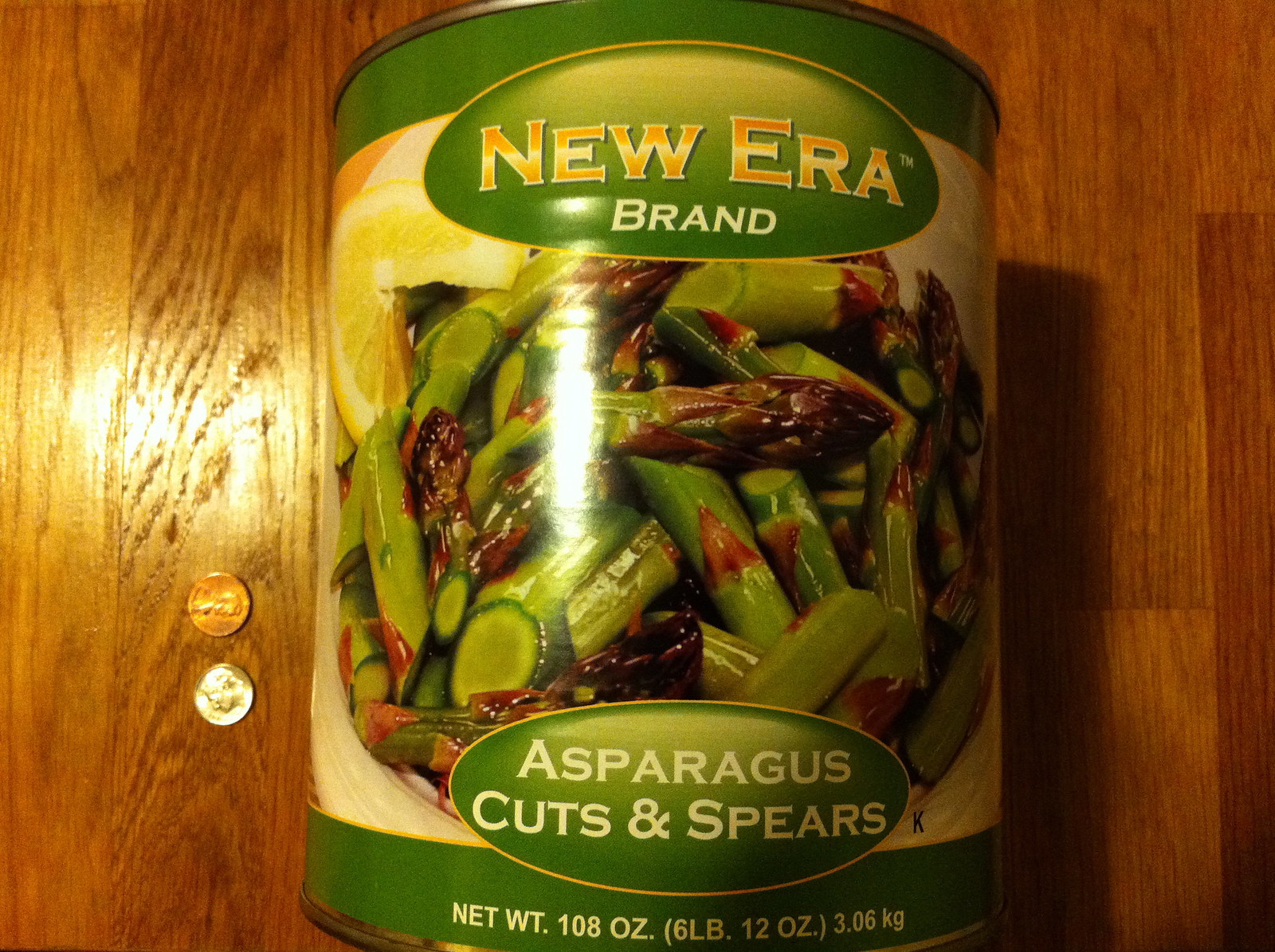Photograph of a can of asparagus resting on a mid-toned blonde-orange table. Two coins are placed next to the can, and light reflections are visible on the table above the coins. The can features a label with a color scheme of green, gold, and white. The brand name, "New Era," is displayed in gold font. The label shows an image of asparagus cuts and spears, some with a brownish hue, accompanied by a lemon slice in the background. The text on the can reads "Asparagus Cuts and Spears" in white font, followed by the net weight details: "108 ounces or 6 pounds 12 ounces or 3.06 kg." Light reflections can also be seen on the can's label.